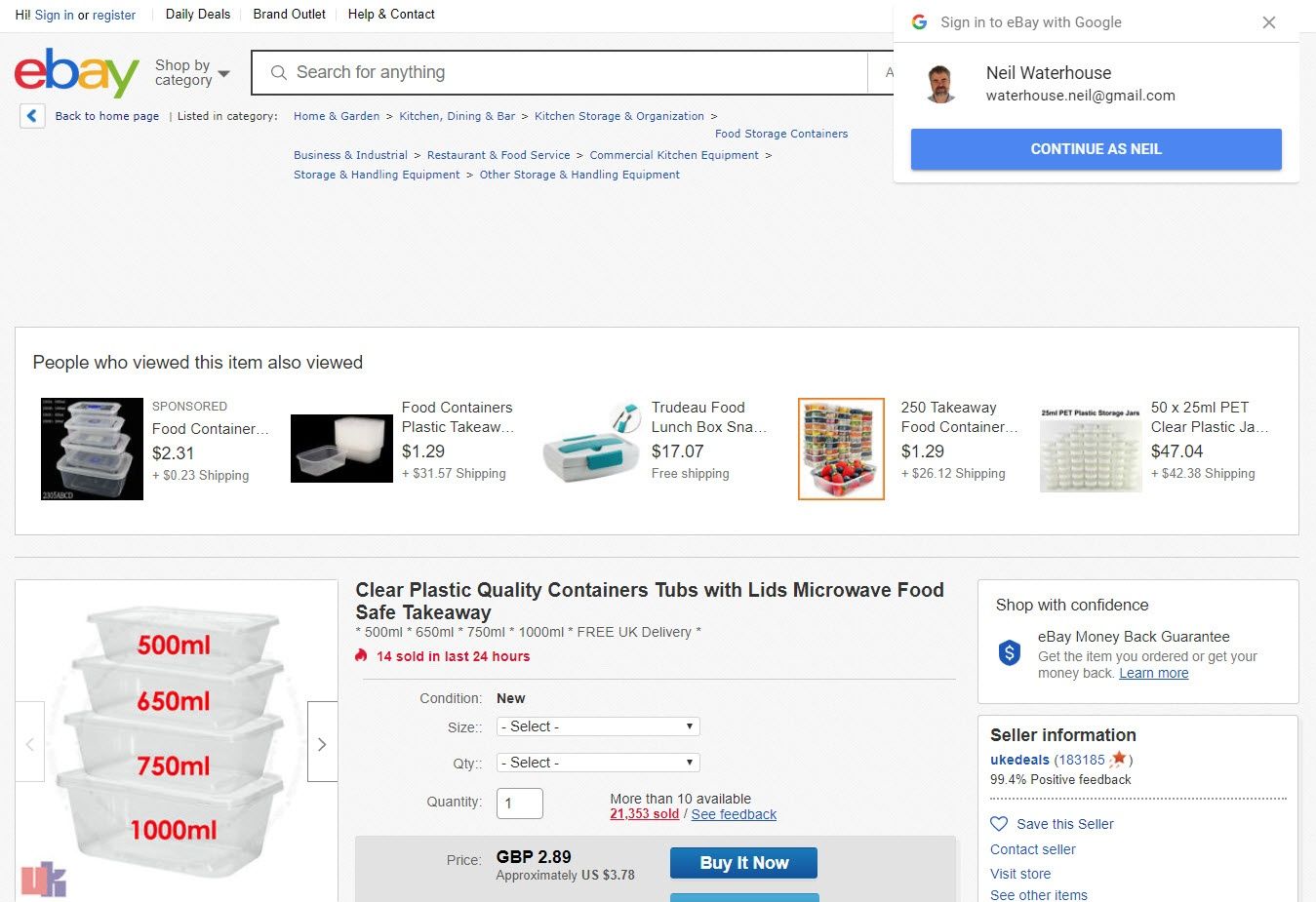This is a detailed screenshot of the eBay website homepage. In the top left corner, the eBay logo is prominently displayed in its signature colors, indicating the recognized brand. Just above the logo, there are user navigation options including "Sign in", "Register", "Daily Deals", "Brand Outlet," and "Help & Contact". The background of the homepage is a light gray color, offering a neutral backdrop to various interface elements.

In the central part of the screen, the user has focused on a particular item. Below the site navigation, a section in a white box is dedicated to "People who viewed this item also viewed," providing suggestions based on the selected item's context. Directly below this, the details of the selected item are displayed including an image of the item, alongside vital information such as the item's name, how many units were sold in the last 24 hours, the condition (new or used), available sizes, quantity, and total available stock. Crucial purchasing options such as the price and "Buy It Now" button are prominently visible. 

To the right of the item details, additional information encourages a secure shopping experience. The “Shop With Confidence” banner highlights the eBay Money Back Guarantee. Below this, there is detailed seller information including the seller's positive feedback percentage, as well as options to save the seller, contact the seller, visit their store, or see other items they have listed.

In the top right-hand corner, an option to sign into eBay using a Google account is available. The person signing in, named Neil Waterhouse, has their email address displayed just below the sign-in prompt, providing a personal touch tailored to the user's account.